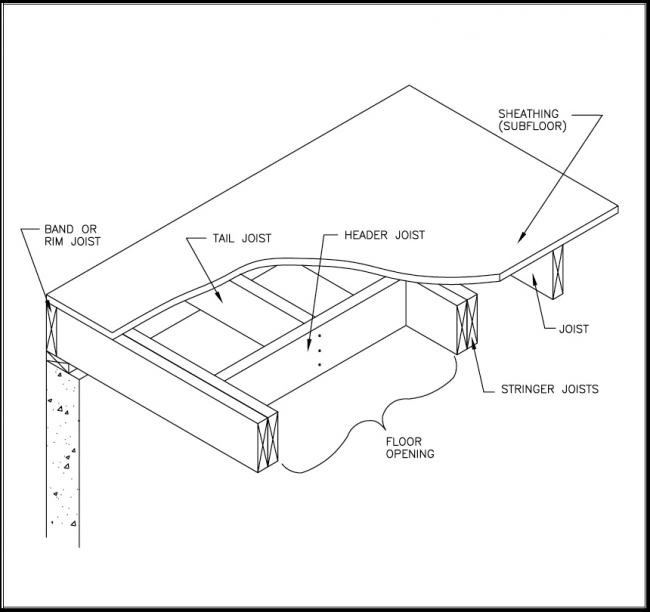This black and white diagram illustrates the construction of a flooring structure, emphasizing various components and their labels. At the top of the image, the flat surface is labeled as "Sheathing Subfloor." Below this, the drawing showcases multiple wooden supports, which are meticulously labeled. To the right, we see annotations for “Joist” and “Stringer Joist,” along with arrows pointing to corresponding blocks of wood. Centrally, the label "Header Joist" is displayed with an arrow pointing to a distinguishable piece of wood marked with three dots. To the left, terms like "Floor Opening" and "Band or Rim Joist" are noted, with an arrow indicating a "Tail Joist." Additional annotations, such as "Floor, Opening," are positioned to the left, tied to specific wooden blocks by arrows. The diagram likely serves as an instructional graphic for constructing a section of flooring, detailing the precise placement and identification of each joist and structural component.